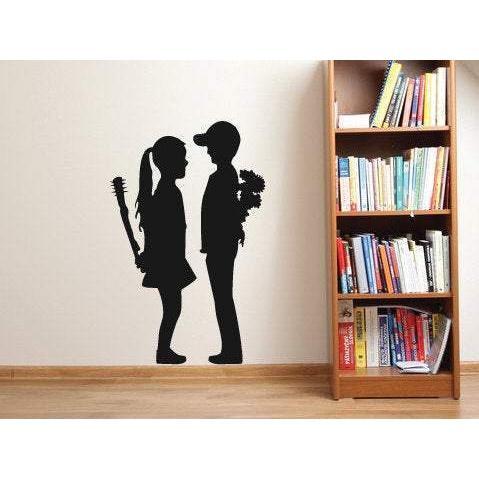The photograph captures an indoor setting, likely a room in a building, featuring a light brown wooden floor that complements the medium brown wooden baseboard. Dominating the right side of the image is a four-tiered bookshelf, filled with books of various colors, suggesting a lived-in and cozy environment. The wall behind the bookshelf is off-white or light gray, creating a neutral backdrop. In the center of the wall are two all-black silhouettes of children positioned facing each other. 

The girl, standing on the left, wears a short dress and shoes, her long ponytail flowing behind her. She holds a stick with nails behind her back, adding an unexpected and edgy element to the scene. The boy, taller and positioned on the right, is dressed in a ball cap, a long-sleeve shirt, pants, and shoes. He holds a bouquet of flowers behind his back, introducing a contrasting gesture of innocence and affection. The silhouettes are meticulously placed just above the wooden baseboard, unifying the aesthetic of the room with this striking decorative element.